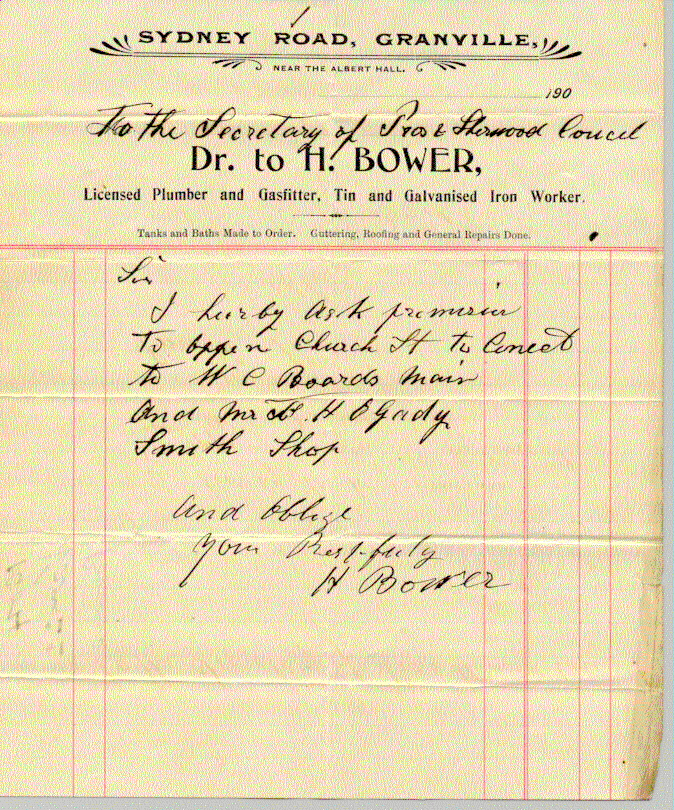This image shows an aged, yellowish piece of paper, possibly a proposal or invoice, featuring both printed and handwritten text. At the top, in black lettering, it states "Sydney Road, Granville, near the Albert Hall," adorned with decorative tassels on both sides. Following that, the number "190" appears in the upper right-hand corner. The document is addressed "To the Secretary of Sherwood Council," followed by "Dr. 2H Bauer." Bauer's credentials are listed as "Licensed Plumber and Gas Fitter, Tin and Galvanized Iron Worker," with additional services noted: "Tanks and Baths Made to Order," "Guttering," "Roofing," and "General Repairs Done." The lower part of the page is lined with red horizontal and vertical lines, likely for itemized entries, and features a section of handwritten cursive text that is largely illegible, though it begins with a formal address "Sir, I hereby ask permission to," and is signed at the bottom by H. Bauer. The overall condition and design elements suggest this is a document from a bygone era.